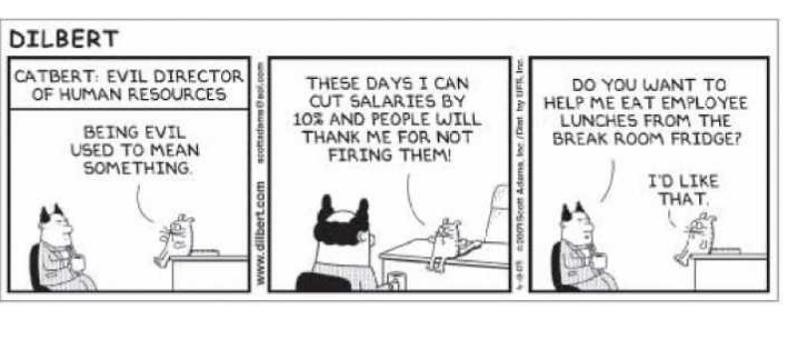This is a three-panel black and white "Dilbert" comic strip, typically found in the comics section of a newspaper. The title "Dilbert" is prominently displayed in bold, capital letters at the top left. The characters include Catbert, the evil director of human resources, and Dilbert, who is seated at a desk with a peculiar hairstyle resembling horns.

In the first panel, the context reads "Catbert, evil director of human resources," and it shows Catbert, a malevolent-looking cat, sitting on a desk. Catbert declares, "Being evil used to mean something." Dilbert, sitting in a black chair nearby, listens with a bemused expression.

The second panel captures Catbert continuing his lament: "These days I can cut salaries by 10% and people will thank me for not firing them." The background remains consistent, emphasizing Catbert's cynical viewpoint.

In the third panel, Dilbert, with his distinctive horn-like hair, responds, "Do you want to help me eat employee lunches from the break room fridge?" Catbert delightfully replies, "I'd like that." Throughout the strip, all text is written in capital letters, enhancing the comic's bold and straightforward style. The web address "www.dilbert.com" appears between the first two panels, and there are some indistinct words between the second and third panels.